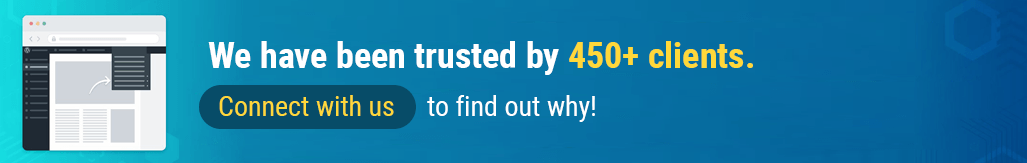Screenshot of a website banner featuring a gradient background that transitions from a neon light blue on the left to a dark navy blue on the right. On the left side of the banner, there's a placeholder layout illustrating blank example boxes where words and infographics would typically appear. Along the right side of this layout, the text reads "We have been trusted by" in white font, followed by "450+ clients" in bold yellow letters. Beneath this, starting from the left, there's a gray box with the message "Connect with us" in the same yellow font. Just outside of this box, the text "to find out why!" is displayed in white letters, encouraging engagement.